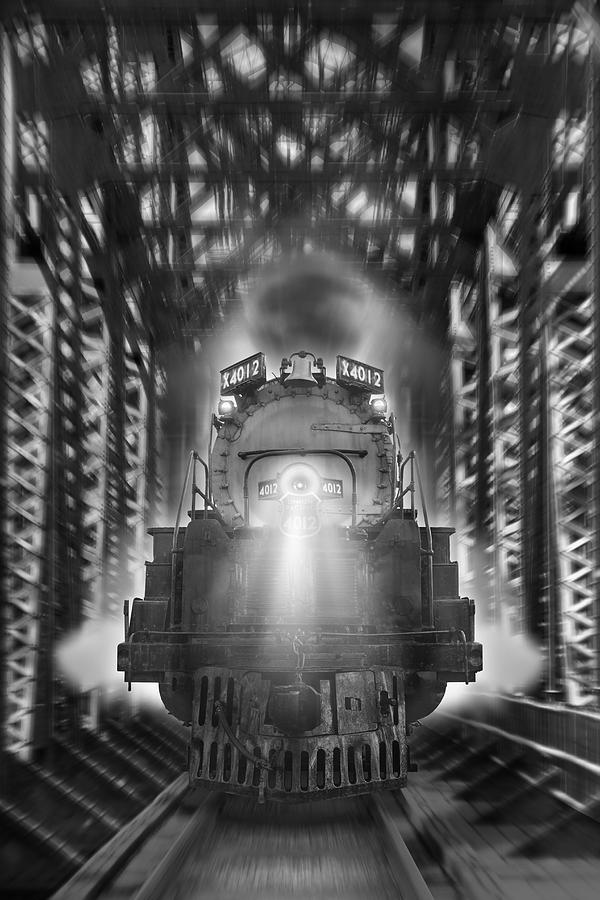The black and white image captures the front view of an old-fashioned steam train, identified by the number X4012 prominently displayed on both the top left and top right corners. The train, which appears to be emitting steam from the sides and smoke from the top, is situated on a railroad track under a metal structure. This structure, supported by zigzag-patterned metal pillars, features a ceiling with a crossed metal pattern. The train's headlight, centered on the front, illuminates the scene slightly. The whole scene is rendered with photographic-like detail, evoking an illustration style. The train is depicted upright within a vertical rectangular frame, and although the wheels aren’t visible, giving an impression of it floating above the tracks, its presence under the metal roof creates a tunnel or covered bridge effect.